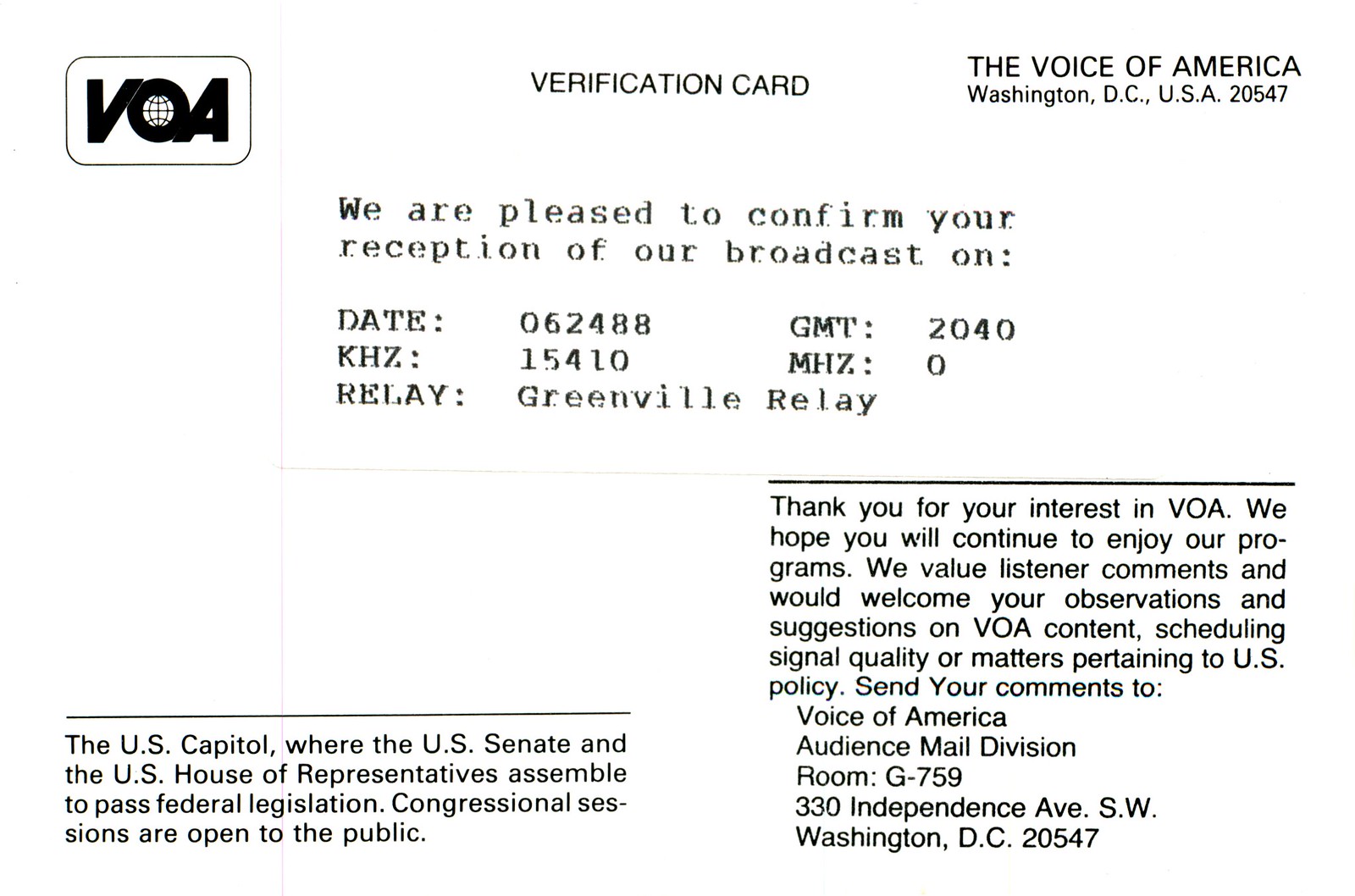The image shows a black-and-white verification card from Voice of America, located in Washington, D.C., USA 20547. The card is in landscape orientation and features black text on a white background. In the upper left corner, there is the VOA logo in bold italics, with the 'O' stylized as a globe. The top center of the card reads "Verification Card," and the upper right corner includes the Voice of America address.

The center of the card contains a block of text confirming broadcast reception: "We are pleased to confirm your reception of our broadcast on Date: 06-24-88, GMT: 2040, KHZ: 15410, Relay: Greenville Relay, MHZ: 0." Below this, two paragraphs are found. The lower right paragraph expresses gratitude: "Thank you for your interest in VOA. We hope you will continue to enjoy our programs. We value listener comments and would welcome your observations and suggestions on VOA content, scheduling, signal quality, or matters pertaining to U.S. policy." The stated contact address is "Voice of America, Audience Mail Division, Room G759330, Independence Avenue, SW, Washington, DC, 20547."

On the lower left, another paragraph describes the U.S. Capitol, where the Senate and House of Representatives pass federal legislation, noting that congressional sessions are open to the public.